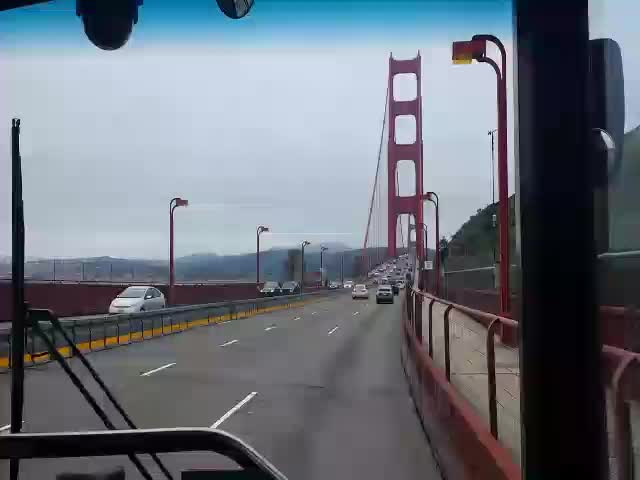This detailed first-person image, likely taken from the front seat of a bus given the expansive windshield, captures the view from a vehicle traveling along the far right lane of a large suspension bridge. The windshield, accompanied by a side window reminiscent of those found in buses, frames the scene. The bridge accommodates three lanes of traffic in each direction, with the mentioned vehicle positioned adjacent to the walkway, separated by a vertical concrete barrier topped with a red railing.

In the distance, approximately 50 to 100 meters ahead, the imposing structure of a vertical suspension bridge pillar is visible. The pillar consists of two vertical legs joined by four horizontal crosspieces at various heights: one near the base, one at mid-height, one higher up, and another at the very top. Suspended from the pinnacle are thick steel cables descending to the roadway, supported further by thinner wires beneath, connected to the bridge's deck.

The background features an overcast sky, casting a gray hue over the entire scene, adding to the dramatic perspective offered by the sweeping view of the expansive bridge and the intricate network of supportive cables.